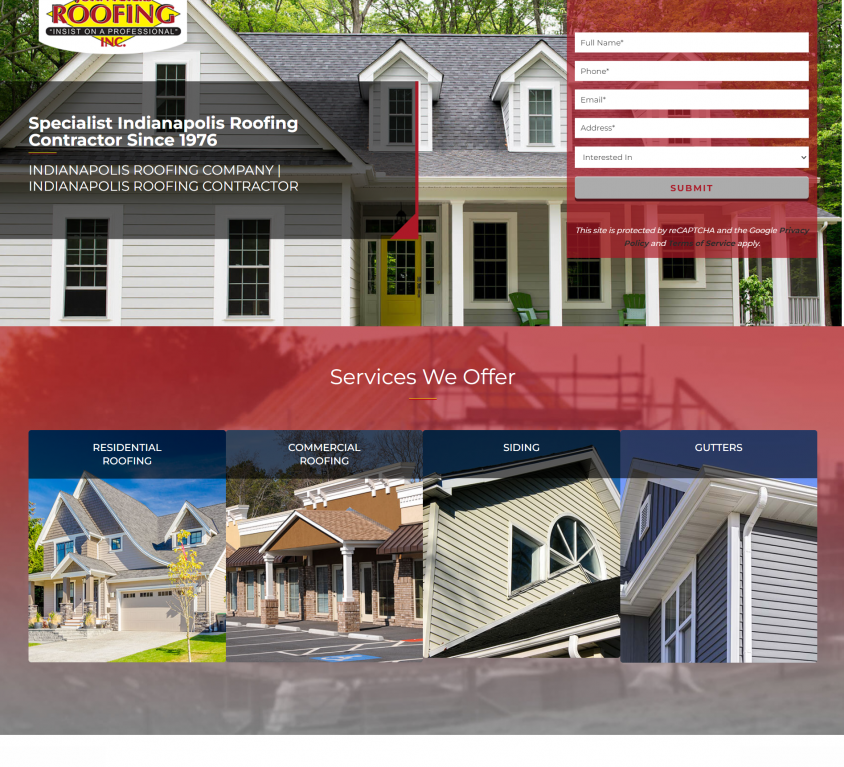This image showcases a webpage designed as an advertisement for a roofing company. Dominating the top left corner of the page is the keyword "Roofing" in prominent text. Beneath it, the term "Owner Profession" is mentioned. 

The background prominently features an image of a white house with a large, standard brick roof. To the right of the page, there is a form that invites users to fill in their full name, phone number, email address, and their specific interest, accompanied by a "Submit" button. 

On the left side of the page, several tabs outline the company's credentials and services:
- "Specialist" 
- "Indianapolis Roofing Contractor Since 1976" 
- "Indianapolis Roofing Company" 
- "Indianapolis Roofing Contractor"

Below these tabs is a red section labeled "Services We Offer." Four distinct pictorial tabs are present in this section:
1. "Residential Roofing" - featuring an image of another house with a gray roof.
2. "Commercial Roofing" - displaying a storefront.
3. "Siding" - showing a gray house and its siding.
4. "Gutters" - highlighting a blue house and its gutters.